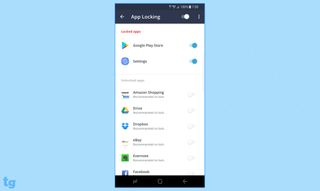This image, categorized under "websites", features a light blue background. In the lower left-hand corner, there are capital letters 'T' and 'G' in a darker shade of blue. The focal point of the image is a phone screen displaying what appears to be an app, likely related to app locking. The main text reads "App Something," possibly indicating app locking functionalities. Just below this text, the Google Play Store logo is visible and marked as "on." Additionally, the "Settings" option is also turned on.

Below these prominent features, there is extremely small text that is not legible. However, one distinguishable icon is the Drive logo, which is shown as "off." In total, there are five or six other app icons listed underneath, all of which are not activated, indicated by their "off" status. Due to the small size of the text and icons, identifying more detailed information is challenging.